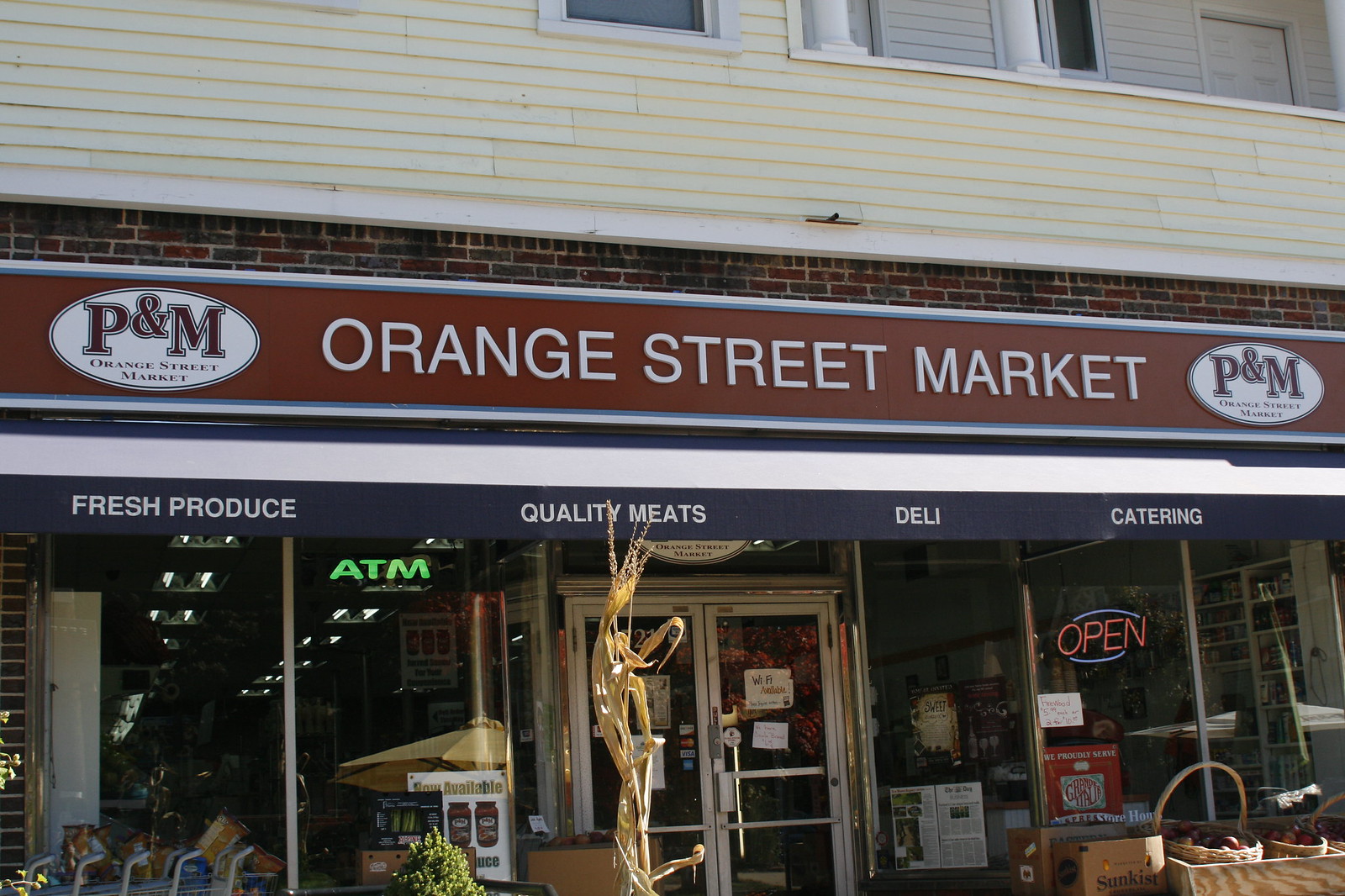The photograph showcases the storefront of the Orange Street Market. Prominently, a red banner with white letters announces the market's name, flanked on either side by circular logos reading "P&M" in red lettering. Below this, a secondary blue banner with white text advertises "Fresh Produce, Quality Meats, Deli, and Catering." The storefront consists of glass windows and doors, the latter featuring metal bars for easy opening and closing. The windows display various food product images and signs. Notably, a neon "Open" sign appears in the right window, while a neon "ATM" sign is evident to the left of the doors. Outside, baskets of fruit, including a significant box of oranges, are arranged in front of the store, adding to its inviting appeal. Above the entire storefront, a portion of the building's brick facade and white siding can also be seen.